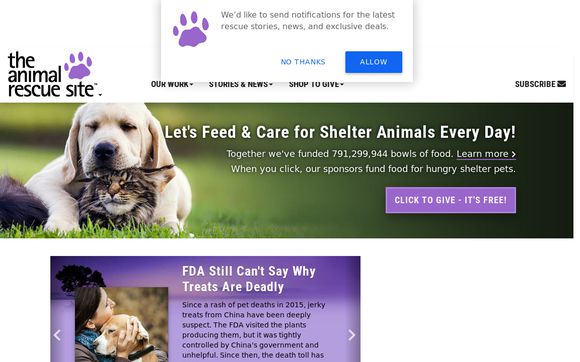**Detailed Caption:**

This screenshot from a website features a predominantly white background. At the top center, a white rectangular pop-up advertisement or menu captures attention. On the left side of the pop-up, there's a purple paw print icon. Adjacent to the icon, black text reads: "We'd like to send notifications for the latest rescue stories, news, and exclusive deals." In the lower left corner of the pop-up, blue text states "No Thanks," while "Allow" is displayed in white font within a purple rectangle.

In the upper left corner of the website, the header "The Animal Rescue Site" is written in black font, accompanied by a purple paw print icon above the word "Site." Further to the right, menu options labeled "Our Work," "Stories and News," and "Shop to Give" are also in black font and designed as drop-down menus. On the far right, the header includes a "Subscribe" option next to an envelope icon, symbolizing email.

Below the header, a graphic bar showcases a heartwarming photo of a yellow Golden Retriever lying in a field, peacefully resting its head on a tabby cat. To the right of this image, a message in white font reads: "Let's feed and care for shelter animals every day."